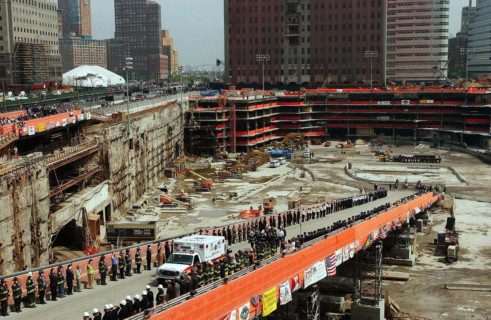This daytime photograph captures a solemn scene at the site of a disaster or demolition area, reminiscent of a ground zero but not located in New York City. In the foreground, a ramp leads from the street into a deeply excavated site, descending five or six stories down. Lined on either side of the ramp, numerous firefighters stand at attention, forming an honor guard as an ambulance ascends from the site, moving towards the street. The image suggests a moment of respect, possibly for remains being respectfully transported away. Skyscrapers and multi-level buildings loom in the distant background, framing the scene with a stark contrast between the city's towering structures and the devastated area below. Among the vehicles, construction equipment is prevalent, indicating active efforts to manage the destruction. An American flag is visible, emphasizing the location within the United States, though the exact site remains unspecified. Onlookers appear to be gathered at the top of the excavation, observing the poignant and busy scene below.